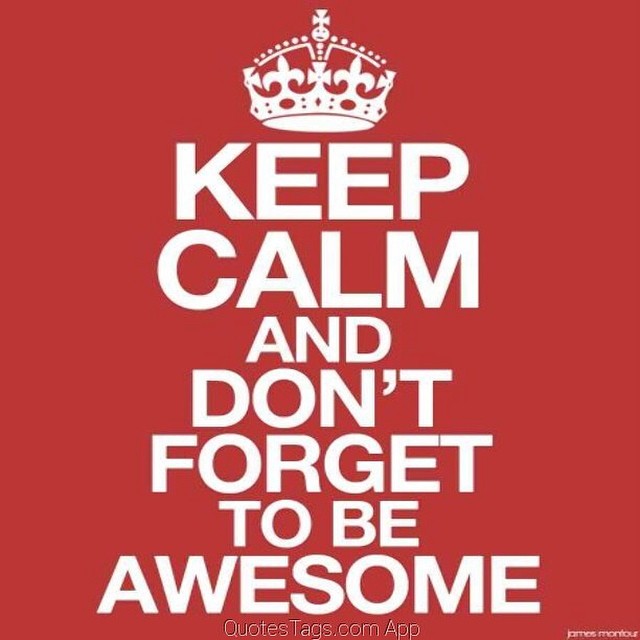The image is a meme with a solid red background and prominent bold white text that reads "KEEP CALM AND DON'T FORGET TO BE AWESOME." At the top, there is a white illustration of a regal British crown, but it features a stern-faced emoji at its center instead of a traditional jewel. Above the crown, a small cross is present. Below the main text, a smaller, thin font with a shadow effect reads "quote tags calm app," indicating likely added text. In the bottom right corner, in a very small and somewhat difficult-to-read font, the name "James Montour" is inscribed, possibly identifying the image's creator. The image shows noticeable JPEG artifacting around the text, suggesting it has been highly compressed.